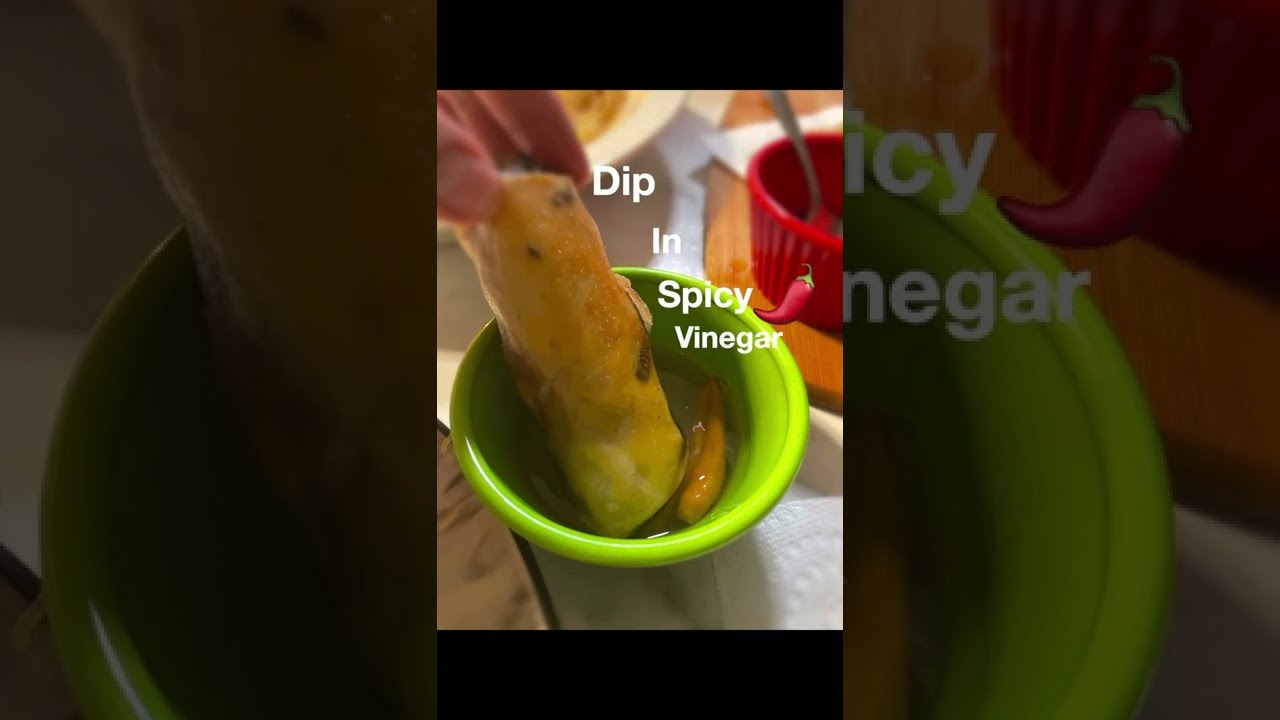The image is a vertical cell phone photo framed with black borders above and below. The scene captures a close-up of a human hand dipping a deep-fried, long food item, possibly a wrapped pastry or burrito, into a small green bowl containing liquid and a green chili pepper. The hand, positioned at the top left, shows the tip of the fingers, thumbnail, and index and middle fingers. Diagonally descending text in white reads "dip in spicy vinegar," accompanied by a red chili pepper emoji next to the word "spicy." The background on the left and right sides features zoomed-in and tinted portions of the central image, with the left side magnifying the left part of the green bowl and the right side focusing on the last three letters of the word "spicy." To the right of the main scene, a red bowl with a spoon rests on a wooden chopping board atop a white tablecloth.